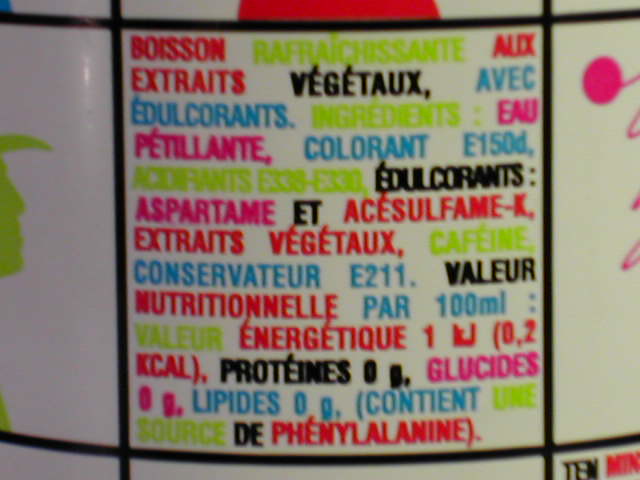The image depicts the back of a white plastic bottle featuring a variety of colorful sections, each containing different images. These sections are distinguished by black lines. One prominent section showcases a multitude of words in various colors—pink, green, blue, and black—written predominantly in French. Although the exact text is not fully decipherable, the language is distinctly French. Surrounding this text section, there are glimpses of other images within the different sections of the bottle, each separated by the aforementioned black lines and varying in color, including notable pink and green shades.